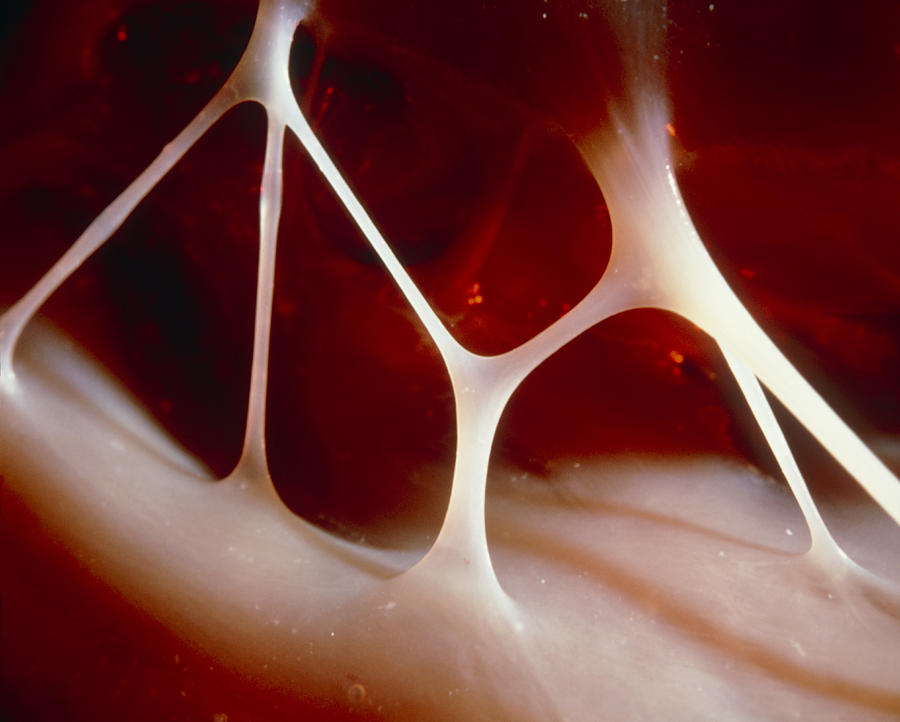In this extreme close-up, we observe a highly detailed and zoomed-in view of what appears to be the inner mouth or throat. Dominated by a pink and red rugged texture that gives the impression of mucous membranes, the background contrasts sharply with lighter areas. Prominently visible at the top of the image is the textured roof of a mouth, from which web-like lines of white, viscous liquid stretch downward. These white membranes resemble sinews or goo, forming rope-like structures that span from the top to a softer, supple structure at the bottom left. The liquid appears thicker near the roof and thins into smaller lines as it descends. The scene is illuminated more brightly from the lower right, casting shadows that deepen towards the upper left and giving the impression of a tunnel-like pathway. The overall scene is relatively clean, devoid of detritus, though with a noticeable dark spot on the left, the origin of which is ambiguous. The intricate and somewhat mysterious biological landscape, with its stretchy and shiny tissues, adds a compelling curiosity to the image.